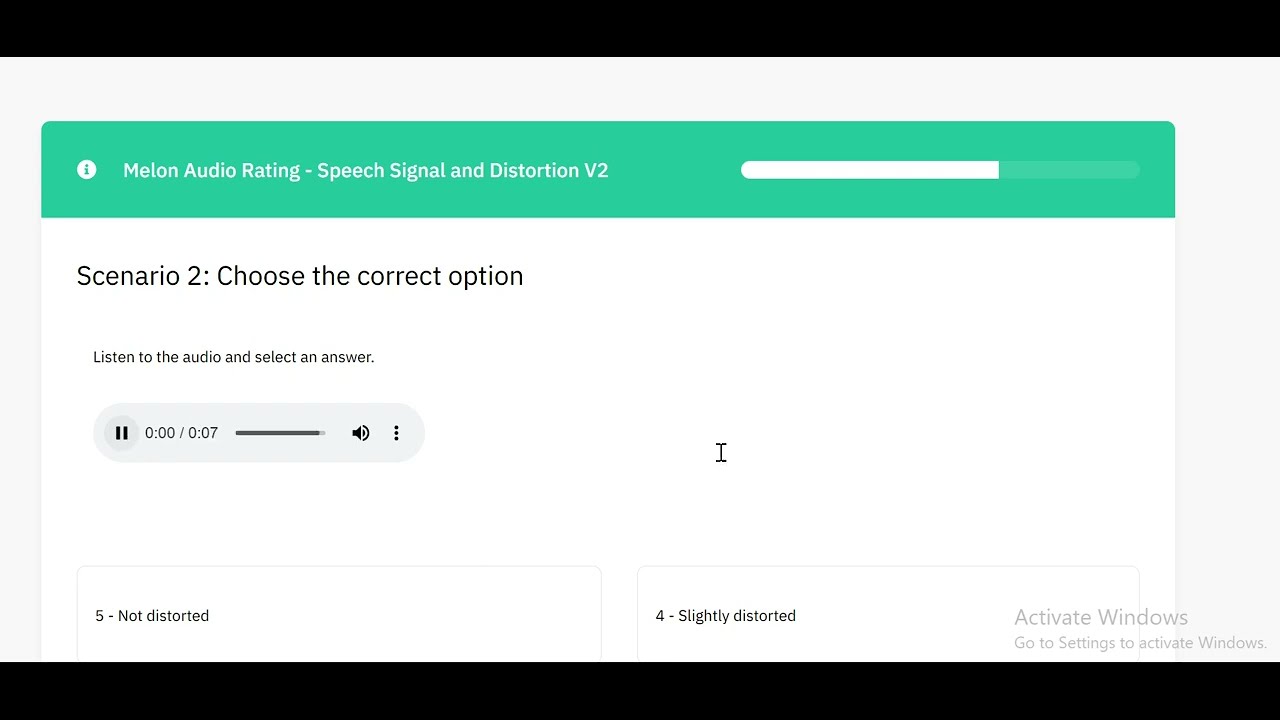The page displays a single question for the "Melon Audio Rating" study. Dominating the top section, a green bar extends across the full width of the page, bearing the title "Melon Audio Rating, Speech Signal, and Distortion V2." Below this header, set against a white background, is the question header, labeled "Scenario 2: Choose the correct option." Underneath this header, smaller text instructs, "Listen to the audio and select an answer."

The page features a standard audio player. On the far left of the player is a pause button, next to which the elapsed time is displayed (currently 0 seconds), followed by a slash, and then the total duration of the audio (7 seconds). Positioned alongside is a longitudinal progress bar that visually represents the playback time. To the right, there is a volume control button, and farther to the right, the player includes a vertical three-dot menu, commonly known as the hamburger menu.

Beneath the audio player, users are presented with response options. "Not Distorted" is labeled as option 5 on the left, and its adjacent option on the right is "4, Slightly Distorted." These are the only two options visible within this frame.